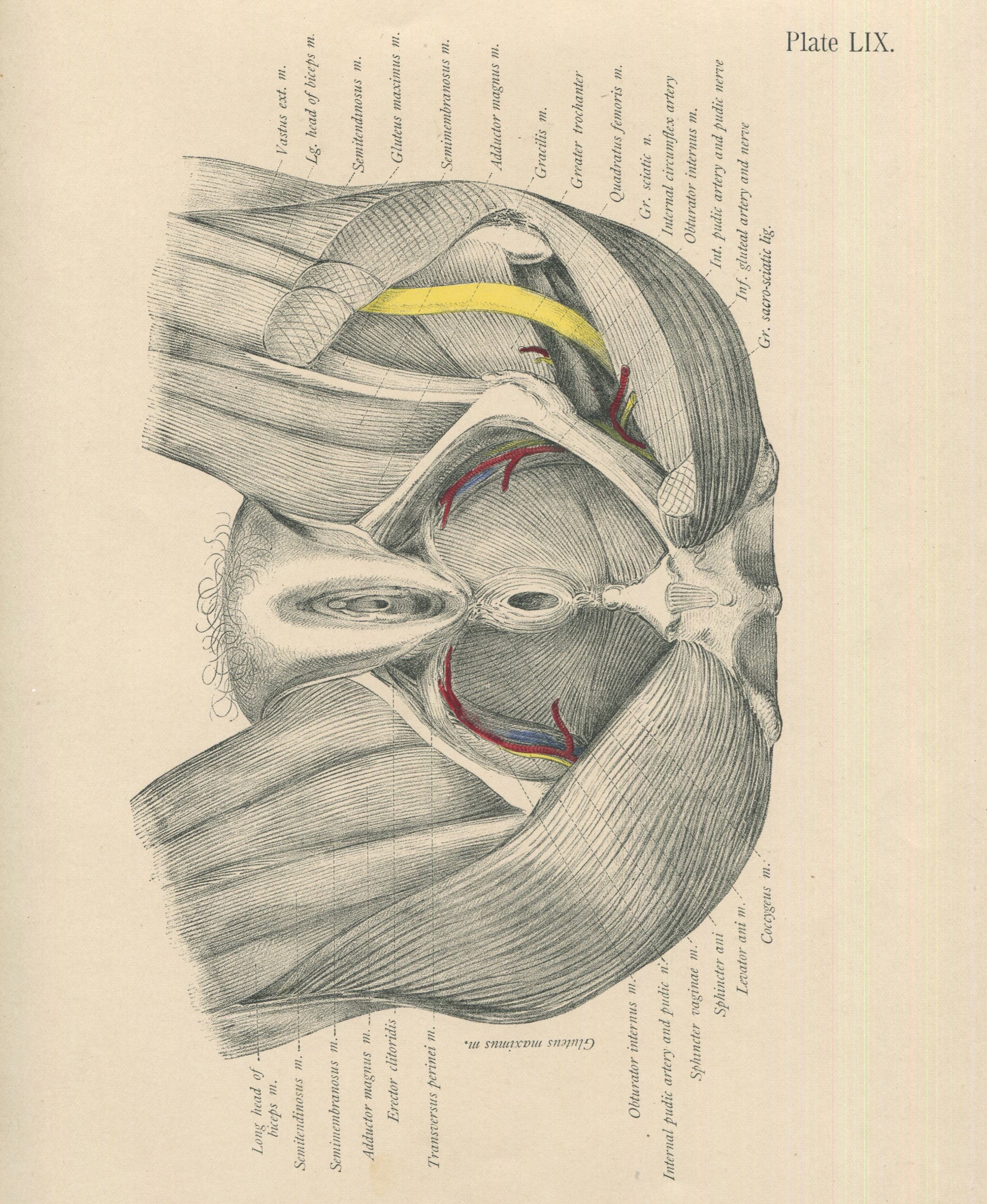This image is an anatomical illustration, likely from a medical textbook, detailing the female genital and surrounding muscular anatomy. The image is drawn in black and white on a light tan parchment-colored background and measures approximately six inches tall by five inches wide. Titled "Plate LIX" in the upper right-hand corner, the piece is viewed sideways, requiring a 90-degree rotation to properly orient. 

At the top of the illustration, two legs are cut off at the beginning of the thighs, revealing the pubic bone with pubic hair in the center between them. The outer vulva and vaginal area are depicted below, with muscles of the buttocks and the anus visible further down. The intricate muscle groups are meticulously labeled on the periphery, using Latin terms that are challenging to pronounce. Notable labels include the "long head of biceps" near the bottom and "transceris peroneal" pointing to an area inside the leg.

The illustration uses minimal color to highlight specific anatomical features: red is used to depict veins around the buttocks, and a yellow strip is shown extending out of the buttocks muscles, possibly representing a tendon. Overall, the image provides a detailed and scientific view of the female lower anatomy, emphasizing the muscle structure and associated parts.